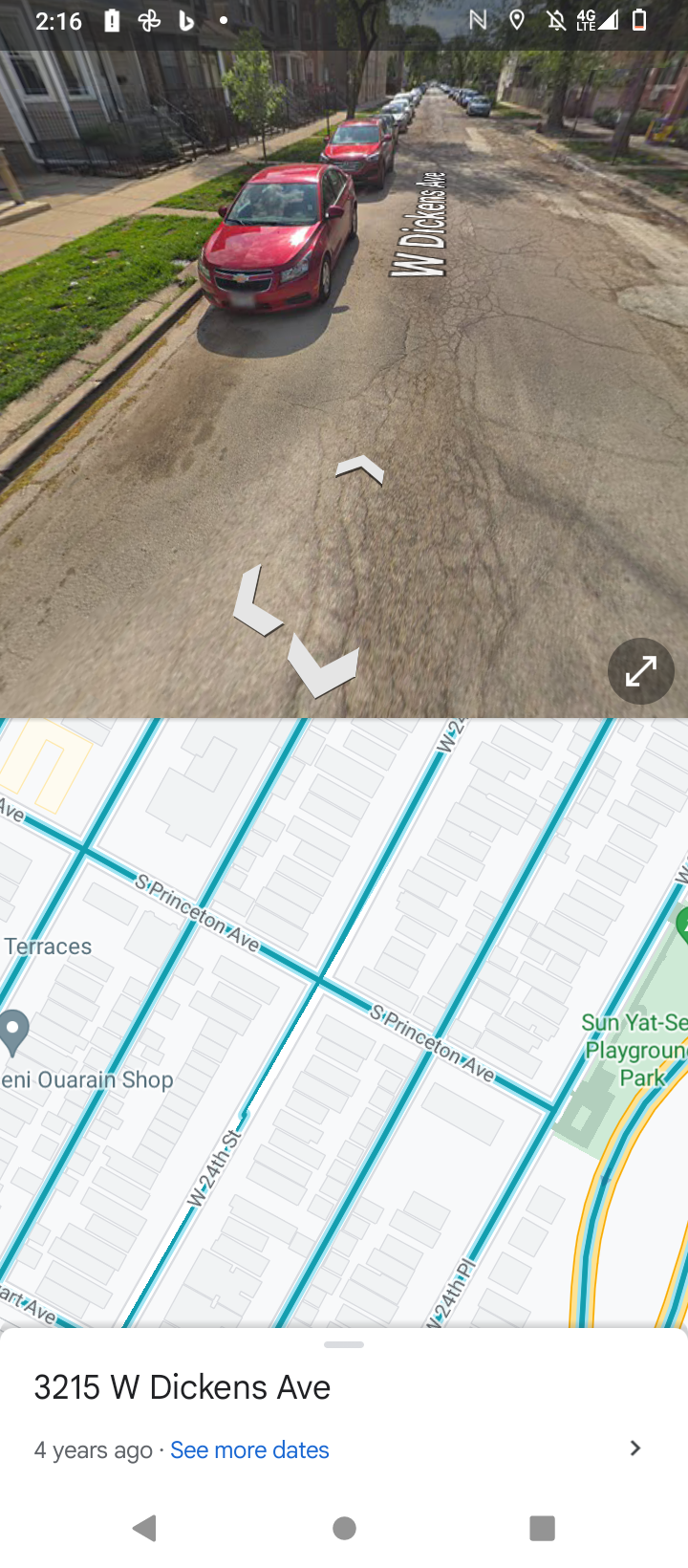This rectangular image is divided into two distinct sections. The bottom half features a Google Maps interface with green lines and labeled locations. The top half showcases a street view, illustrating a road lined with parked cars on the left-hand side. Prominently, two red cars are visible, with additional, less distinct cars trailing behind them. Adjacent to the road, there is a sidewalk bordered by a grassy strip. Scattered trees are planted on both sides of the street, contributing to the suburban ambience.

On the left edge of the image, part of a house or residential building is visible. The road itself displays typical Google Maps features such as directional arrows pointing up, down, and to the left, along with a partially obscured "W" marking, likely indicative of the street name. Additionally, further down on the right side of the street view, there is an interactive double-headed arrow, allowing for navigation within the map. The specific address highlighted in this view is 3215 West Dickens Ave.